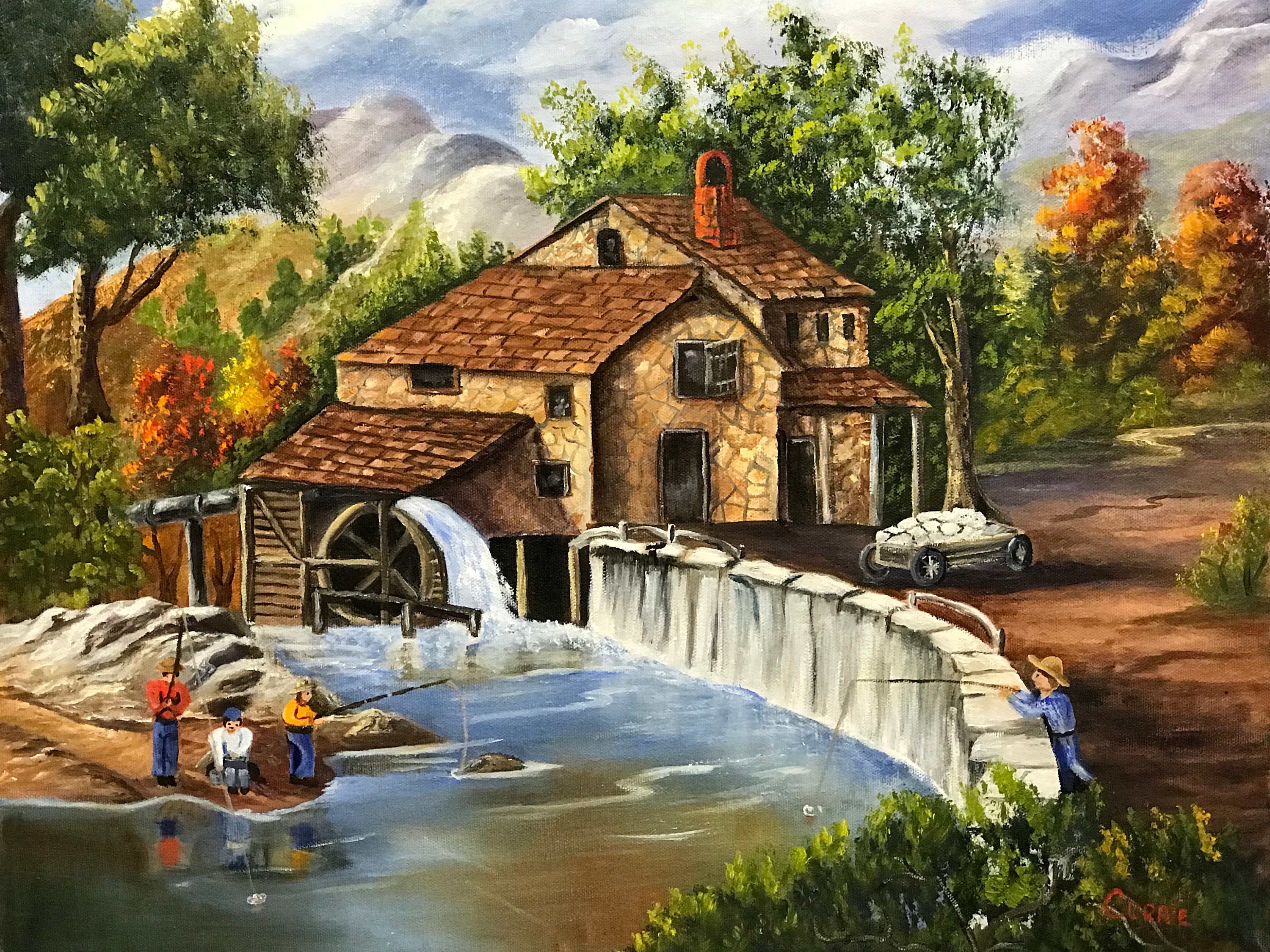The painting, done in a style reminiscent of Thomas Kinkade, features a serene country scene centered around a charming stone country house with a brown roof and a red chimney. The house, which has two separate doorways with one set under a porch and several small windows, is flanked by a water wheel on its left side that feeds into a flowing river. To the right, a dirt driveway leads past a stone wall. By the wall, a boy wearing blue clothing and a brown straw hat is fishing.

Closer to the foreground on the left bank of the water, brush is depicted while three individuals, adorned in red, white, and orange shirts with blue pants, are also fishing. Behind them, rocks and trees serve as natural backdrops. The trees, adorned in the warm hues of fall—red, yellow, and green—frame the scene, while distant mountains peek out on the horizon under a partially visible blue sky with clouds.

Additional details include a fence running alongside the house and a cart filled with sacks on the dirt road. The artwork also features a subtle red signature, possibly "Claire," tucked in the bottom right corner, partially obscured by a bush. The meticulous composition captures a quintessential autumn day with a tranquil, almost nostalgic atmosphere.